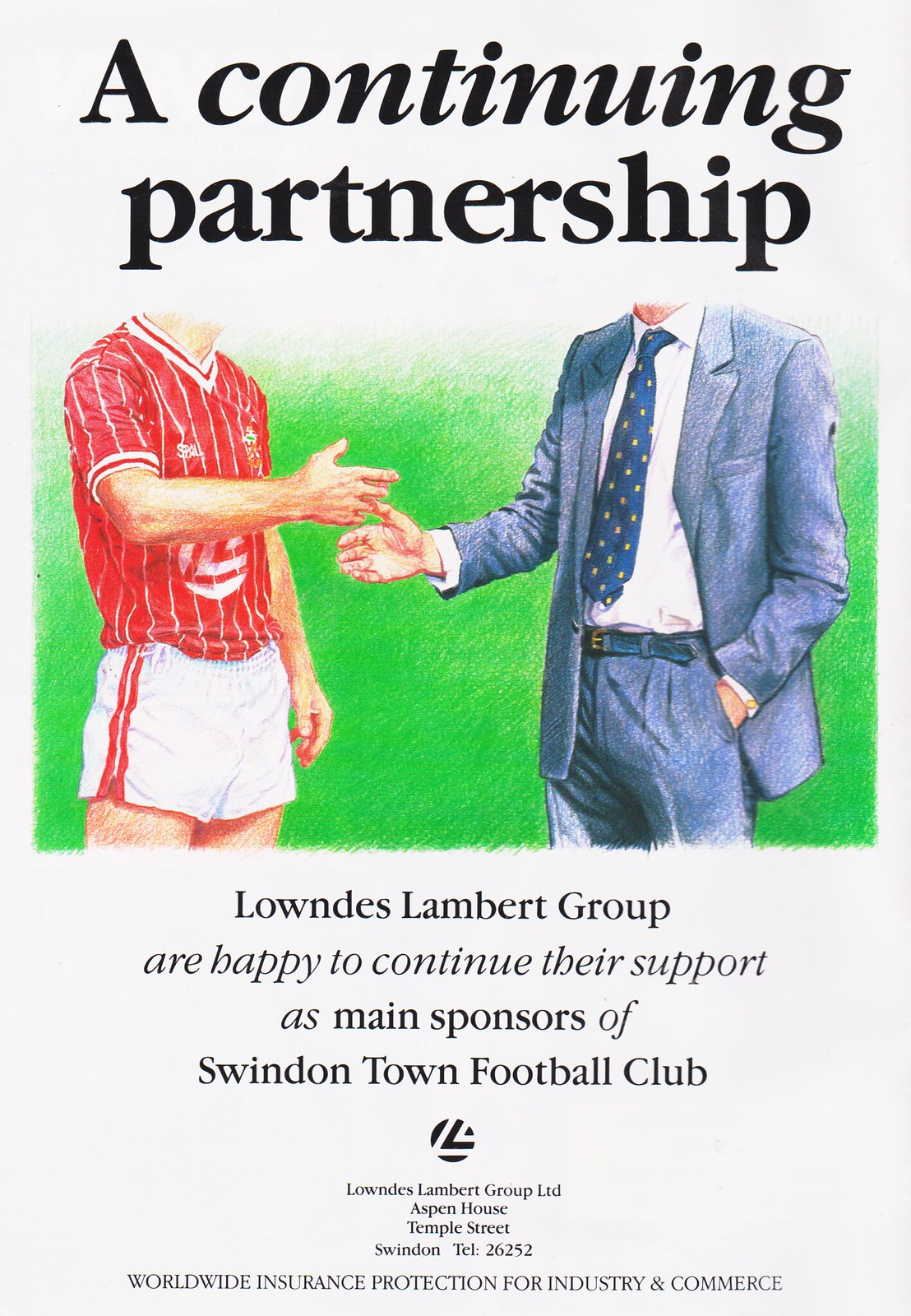This image resembles an old-time advertisement for a football club, prominently showcasing a continuing partnership between a business and a sports team. The artwork depicts the bottom halves of two headless figures in the center. On the left, there is a soccer player wearing a red shirt with white vertical stripes and white shorts, poised to shake hands. On the right, a business person dressed in a full blue business suit, with a white dress shirt and blue tie, is extending his right hand for a handshake, while his left hand is tucked into his pocket. Both figures stand on a green soccer field set against a white background.

Above them, in bold black letters, the text reads: "A Continuing Partnership." Below, it states, "Lowndes-Lambert Group are happy to continue their support as main sponsors of Swindon Town Football Club." Further down, it notes that the sponsorship is by "Worldwide Insurance Protection for Industry and Commerce." This image exemplifies a business's declaration of ongoing sponsorship for a local football club, fostering a positive and supportive relationship.